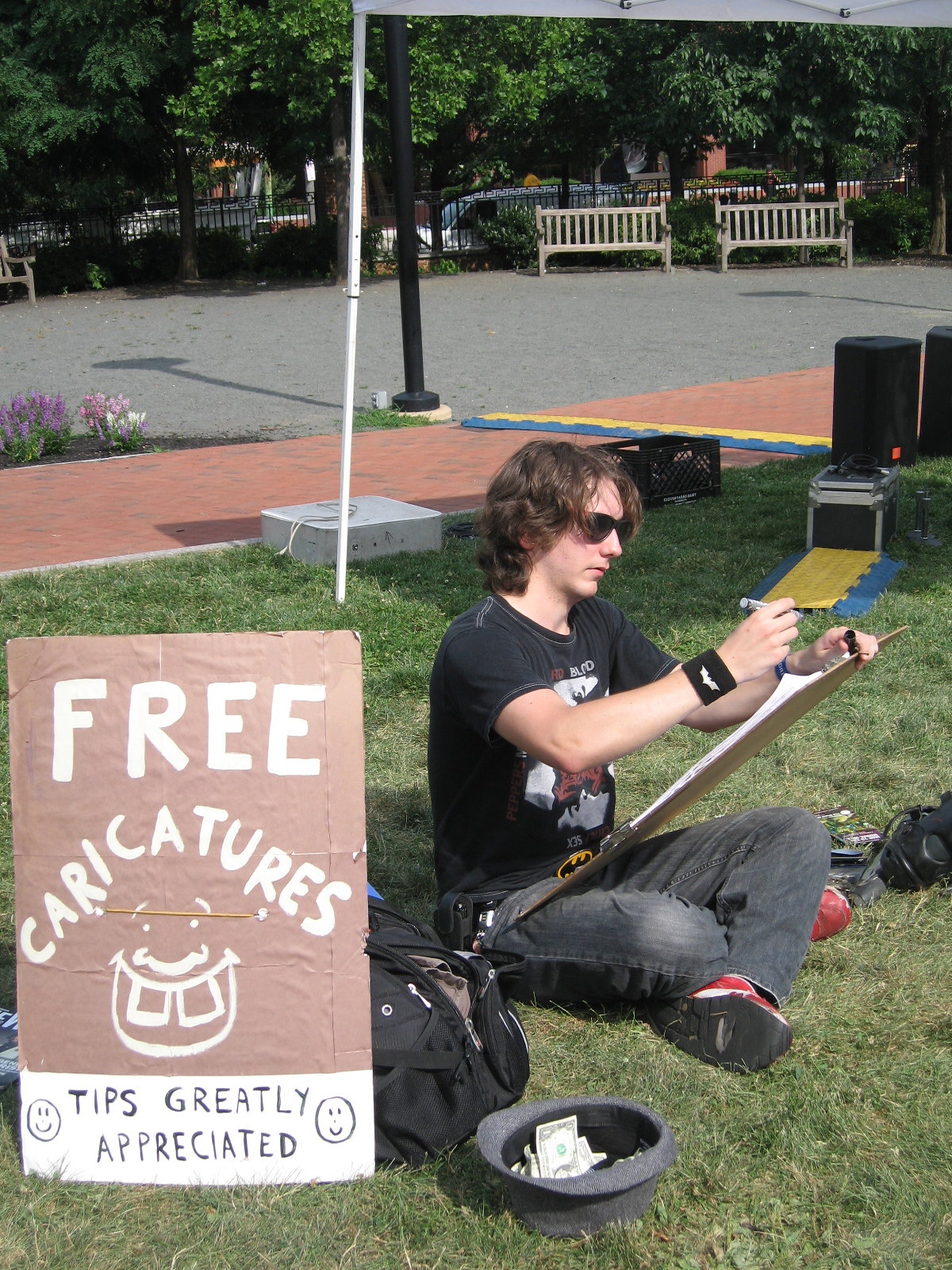In a vertical photograph taken on a sunny day, a young artist is seen sitting crisscross applesauce on the grass in a park. Dressed in a black t-shirt, black jeans, and red shoes, the artist is actively drawing on a clipboard held in one hand with a marker. Beside him is a large sign with a brown top section that states "Free Caricatures" in white lettering, and a white bottom section that reads "Tips Greatly Appreciated" in black lettering, adorned with smiley faces on either side. Near him is a hat placed upside down with some money inside, used for collecting tips, along with a small bucket. The backdrop features a sidewalk, a street, park benches, a lamppost, and various trees, all basking in sunlight. Although the artist is focused on his work, the person he is presumably drawing is not visible in the image. Additional details include a Batman belt buckle and wristband, alongside a bag resting next to him. There are no other people present in the immediate vicinity of the photograph.